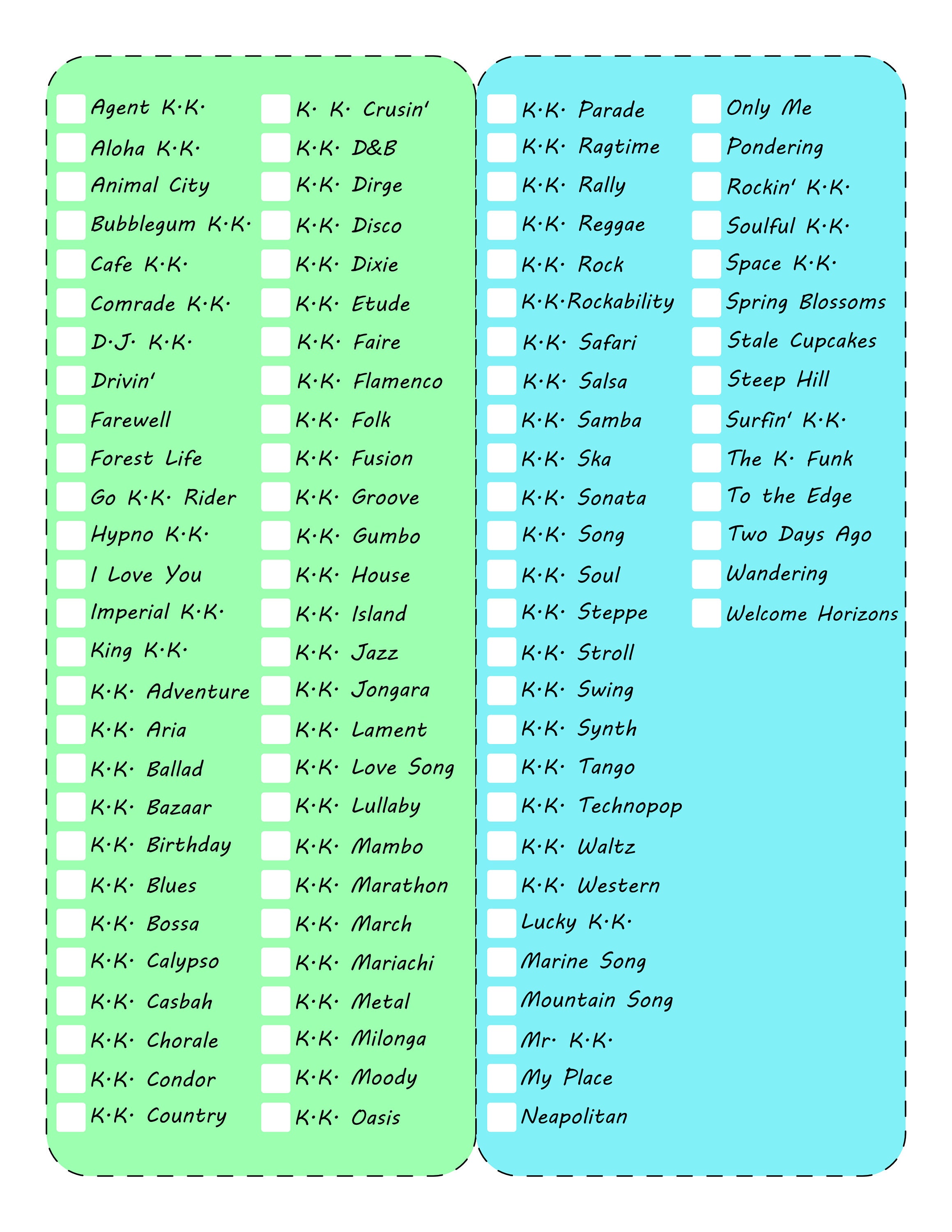The image depicts two vertically aligned checklists of KK Slider songs, each encompassing a range of song titles. The checklist on the left is set against a lime green background, while the one on the right has a seafoam blue background. Both checklists are well-lit, making the black text easily readable. Each list features two columns of song titles that start with "KK" or end with "KK." For instance, the green list begins with "Agent KK" and includes titles like "KK Cruisin'," covering songs alphabetically up to "Oasis." The blue list starts with "KK Parade" and includes entries such as "KK Ragtime" and "Welcome Horizons," arranged alphabetically. These checklists are designed to be printable and are available in JPG and PDF formats. The columns are populated with familiar KK Slider songs like "Farewell," "Blues," "Mambo," "Groove," "Disco," "Reggae," "Samba," "Waltz," and "Western," offering a comprehensive collection for fans.